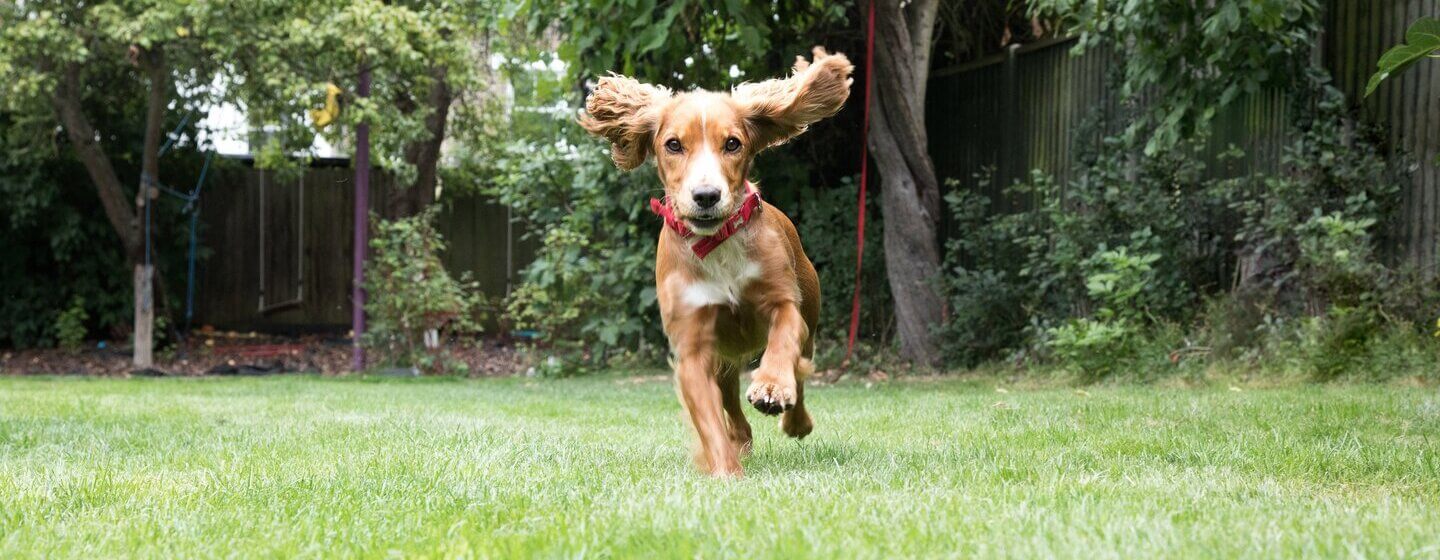In this high-resolution, wide-angle photograph, we see a playful, light brown and white puppy at the center, captured mid-run towards the camera. The adorable medium-sized dog, wearing a red collar possibly attached to a faint red cord in the background, features large, fluffy ears suspended in the air, highlighting its swift motion. His expressive eyes gaze directly into the camera, with two paws in the air and two on the well-manicured grass of a medium-sized backyard. The scene is framed by wooden fencing on both sides, with various small trees, shrubs, and a set of wooden swings near the fence, creating a cozy and vibrant atmosphere. The backyard’s landscape includes a notable blend of greenery, accentuating the lively spirit of the moment.